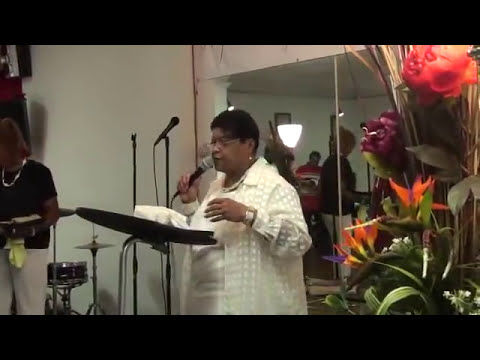In the image, an older black woman, likely in her 50s or 60s, is giving a speech or possibly singing, holding a black microphone in her hand. She is slightly overweight, with short black hair and glasses, and is dressed in a white vest over a white dress. She stands before a black podium adorned with some white materials. Off to her left, another woman, wearing a black top and white pants, holds what appears to be a Bible, suggesting a church setting. A drum set is partially visible near her. On the right side of the image, there is a vibrant bouquet of orange, red, and purple flowers with green leaves. Behind the speaker, a large mirror mounted on the white wall reflects several people standing in the room, adding depth to the scene. The room is filled with various colors including red, purple, orange, yellow, green, black, white, brown, and silver. The overall setup of the image, with the podium and the speaker at the center, surrounded by other details, creates a focused yet lively atmosphere.